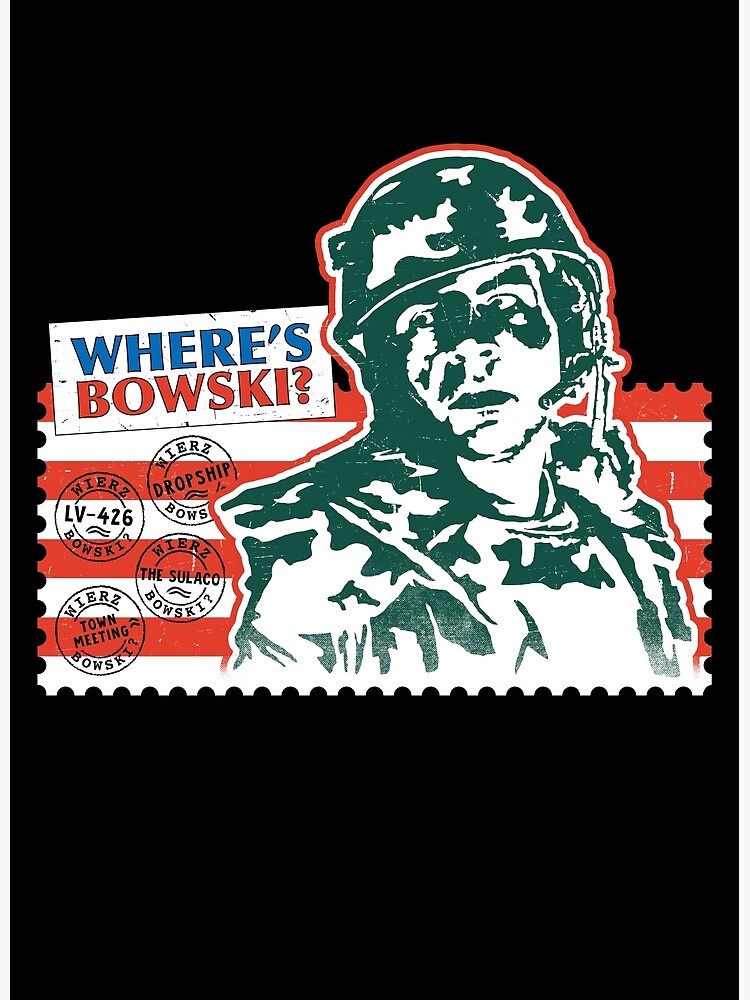The image features a black background with a white rectangular text box at the top, containing the phrase "WHERE'S BOESKY?" The word "WHERE'S" is rendered in blue, while "BOESKY" is in red, both in all capital letters and utilizing a large font size reminiscent of the "Where's Waldo" style. Beneath the text, the background is adorned with red and white stripes, evoking a postage stamp aesthetic. An illustration of a soldier, depicted in green, occupies the center-right of the image. The soldier wears a circular green helmet with white splotch marks, a chin strap, and a green military outfit with visible lines under his eyes. On his shoulders, he has green-colored patches. Several stamp-like markings are superimposed on the red and white stripes, bearing the text "Mirrors Dropship LV-426 Town Melting" and "Sulaco," which suggests a military theme.